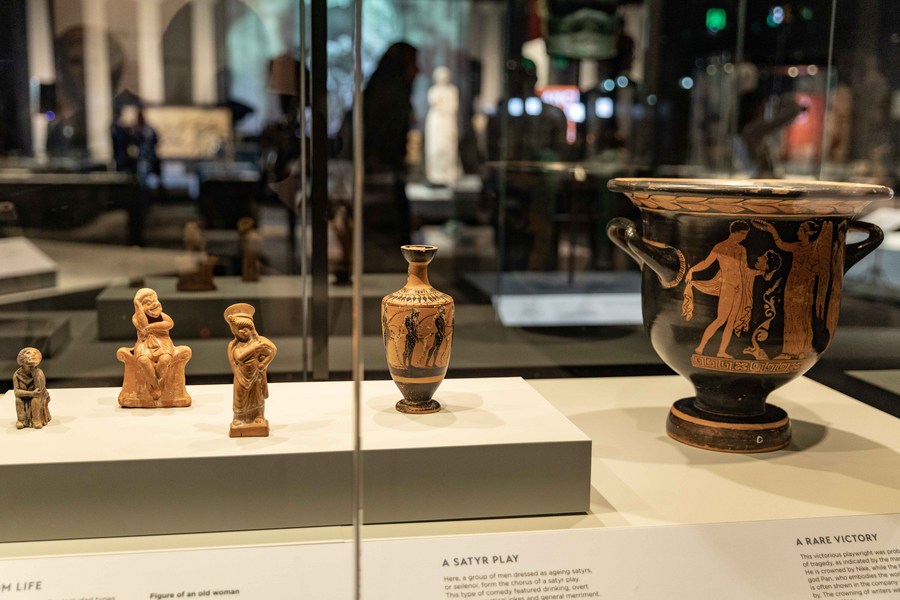This color photograph captures a detailed and vivid scene of an art exhibit showcasing Egyptian and Greek-influenced pottery and sculptures encased in a large glass museum display. On the far right, there is a prominent black pot adorned with bronze figures, notably a man holding a severed head with two angelic figures to his right. This pot is intriguingly titled "A Rare Victory." To its left, there is a smaller pot named "A Satyr Play," featuring several bronze men standing side by side, with black accents on its base and tip. Adjacent to these vases, there are three smaller bronze-colored human figures: one standing, one seated on a chair, and one on a stool, with the leftmost figure exhibiting a bronze-black coloration.

The display case also contains a small sculpture of a squatting person on the left end, possibly indicative of Greek influence. Above or near the "A Satyr Play" pot is a placard that reads: "A Satyr Play. Here, a group of men dressed as aging satyrs or selenoi from the chorus of a satyr play. This type of comedy featured drinking," though the text becomes illegible beyond that point. In the blurred and active background, reflections in the glass case reveal museum visitors walking and examining other exhibits, enhancing the lively and immersive atmosphere of the museum setting.